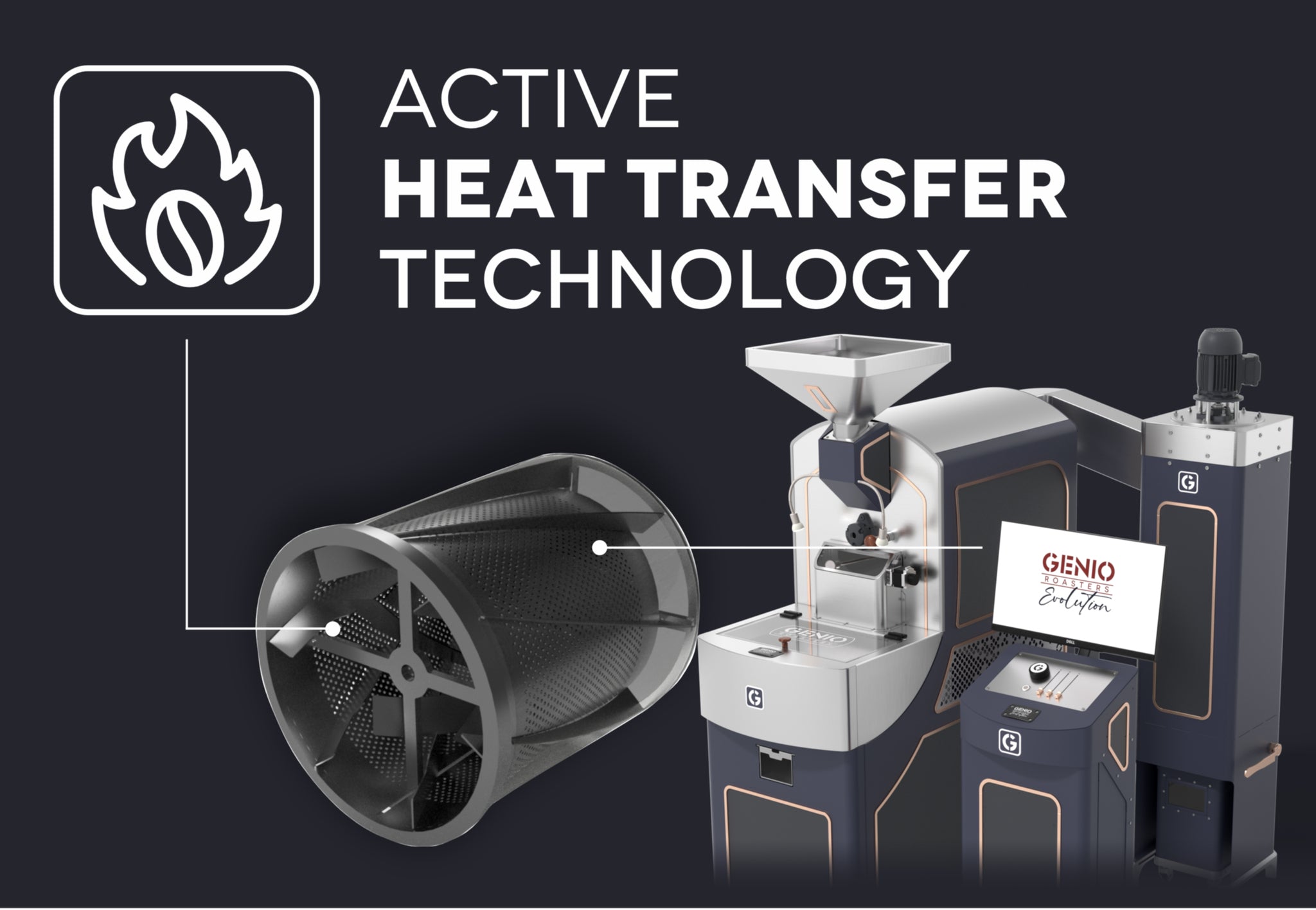The image appears to be an advertisement featuring a sophisticated coffee roasting machine set against a dark gray, metallic charcoal background. Central to the image is the machine itself, which is predominantly gray and blue and composed of two distinct towers. One tower houses the control panels, while the other seems to be where the coffee beans are placed for roasting. On the left side of the image, a rounded square icon with a flame inside, crossed by a circle and a cross, is displayed, highlighting the machine's 'Active Heat Transfer Technology.' Adjacent to the flame icon is text in white font that reads “Active Heat Transfer Technology.” Additionally, the branding and logo are situated on the right side, clearly displaying "Genio Evolution" and "Roasters" in white. The image emphasizes the advanced heat transfer mechanisms and the modern design of the coffee roaster, hinting at its efficient and innovative roasting capabilities.